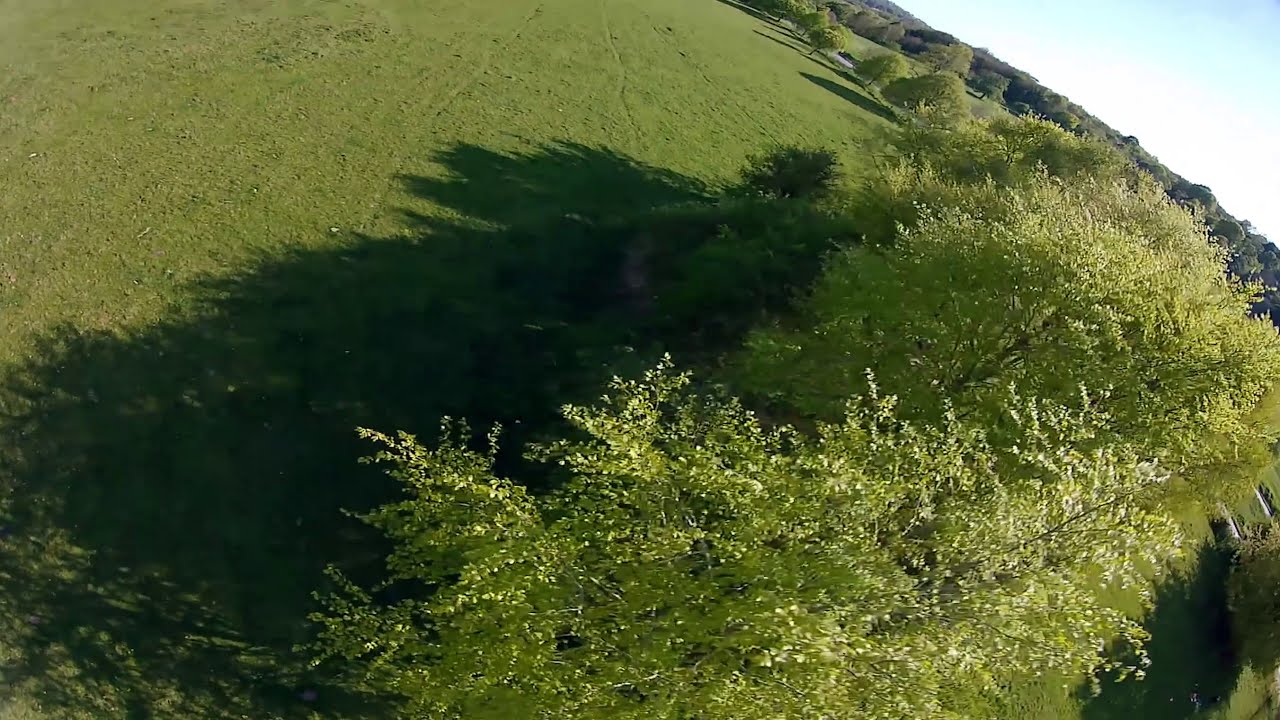This image, likely taken from a drone or GoPro, captures a vibrant grassland scene tilted slightly to the right, presenting a unique perspective. The lush grass, predominantly on the left side, contrasts with a row of verdant deciduous trees on the right. These trees, appearing lighter green with occasional white wisps, extend towards the background, diminishing in size and density to create a sense of depth. The top right corner features a clear blue sky tinged with white, bordered by a distant assembly of trees. Shadows cast by the trees stretch across the central grassland, adding depth and texture. The image's angle and slight distortion emphasize the interplay between the green expanse and the sky, creating an engaging visual experience.